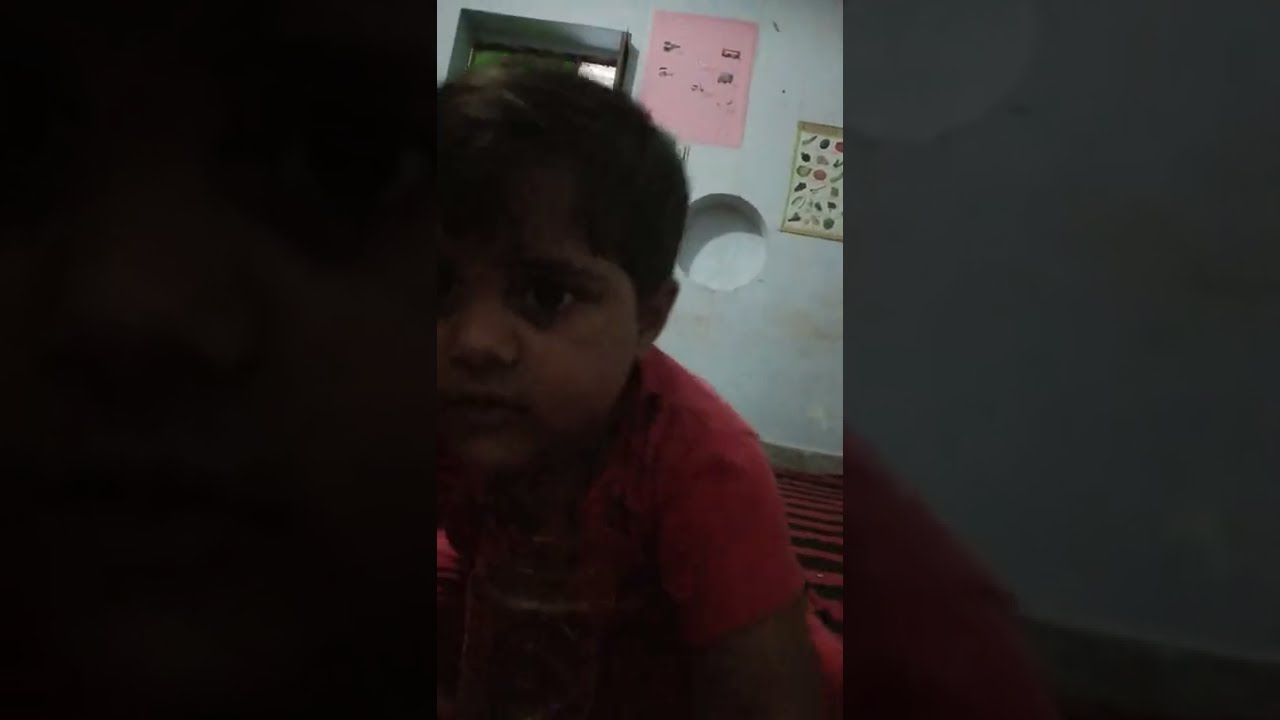The image is a wide rectangular photograph that is divided into three distinct sections. The first section on the left is a solid black rectangle. The middle section features a young boy, possibly of Middle Eastern descent, with darker-toned skin, short dark hair, and large dark eyes. He is wearing a red t-shirt and occupies the central space, with half of his face obscured. Seemingly covering the left side and diagonally extending to the right, this part is well-lit and detailed. The background suggests he’s in a room with a reddish-black striped rug, a white wall adorned with a couple of pictures—one being a chart that's hard to decipher, and what appears to be a mirror right behind his head, showing a hint of sunlight or reflection with a black frame. Additionally, there is a round hole in the wall that resembles a shelf, next to which is a piece of artwork depicting various objects, and above it, a pink poster. A window also appears to be part of the background. The right section of the image consists of a grayish close-up of the child's shoulder against a black background, making this side appear more fragmented and dark.